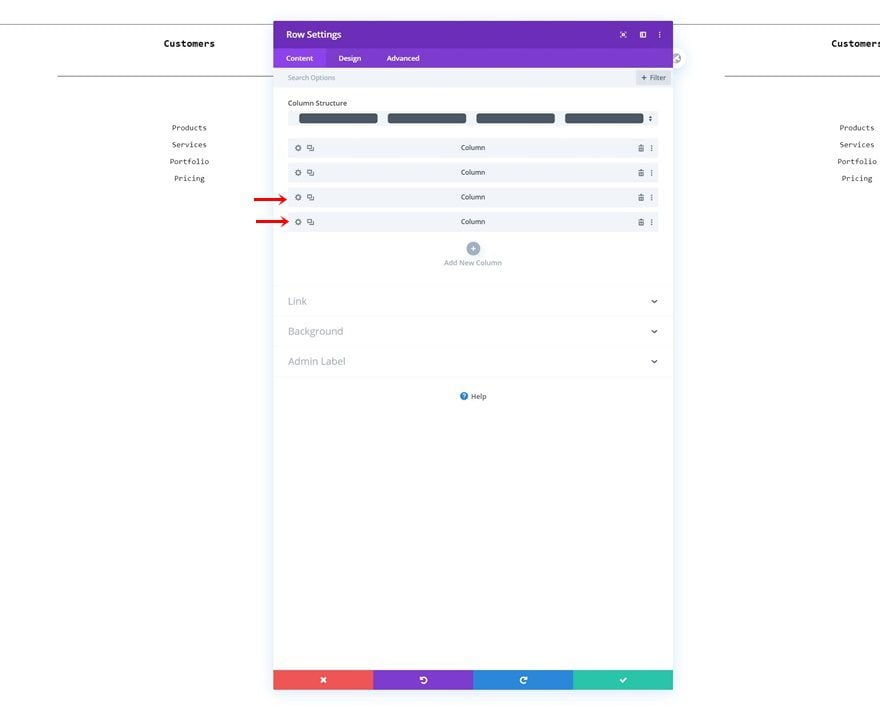A detailed screenshot in landscape mode captures a portion of a user interface, evident by a prominent pop-up message obscuring the central background. In the upper left-hand corner of the underlying content, a bolded text reads "Customers" with a corresponding "Customers" label mirrored on the far right end of the row. Below the "Customers" label on both sides, there are aligned columns listing "Products," "Services," "Portfolio," and "Pricing."

The central portion of the screenshot showcases a purple header labeled "Row Settings." Directly beneath this header, the menu displays "Content, Design, Advanced," with "Content" being currently highlighted. Following this, a row labeled "Search Options" appears, featuring a button marked "Plus Filter" on the far right side. Below this, a section titled "Column Structure" is visible, containing four black rectangles that seem intentionally blacked out.

The user appears to have highlighted the last two entries in the column structure with red arrows, drawing attention to them; however, the heavy redactions make it unclear what changes or additions are being suggested. Additionally, toward the bottom of the screen, the faint text reads "Link Background Admin Label," almost blending into the white background due to its very light gray color, making it difficult to decipher.